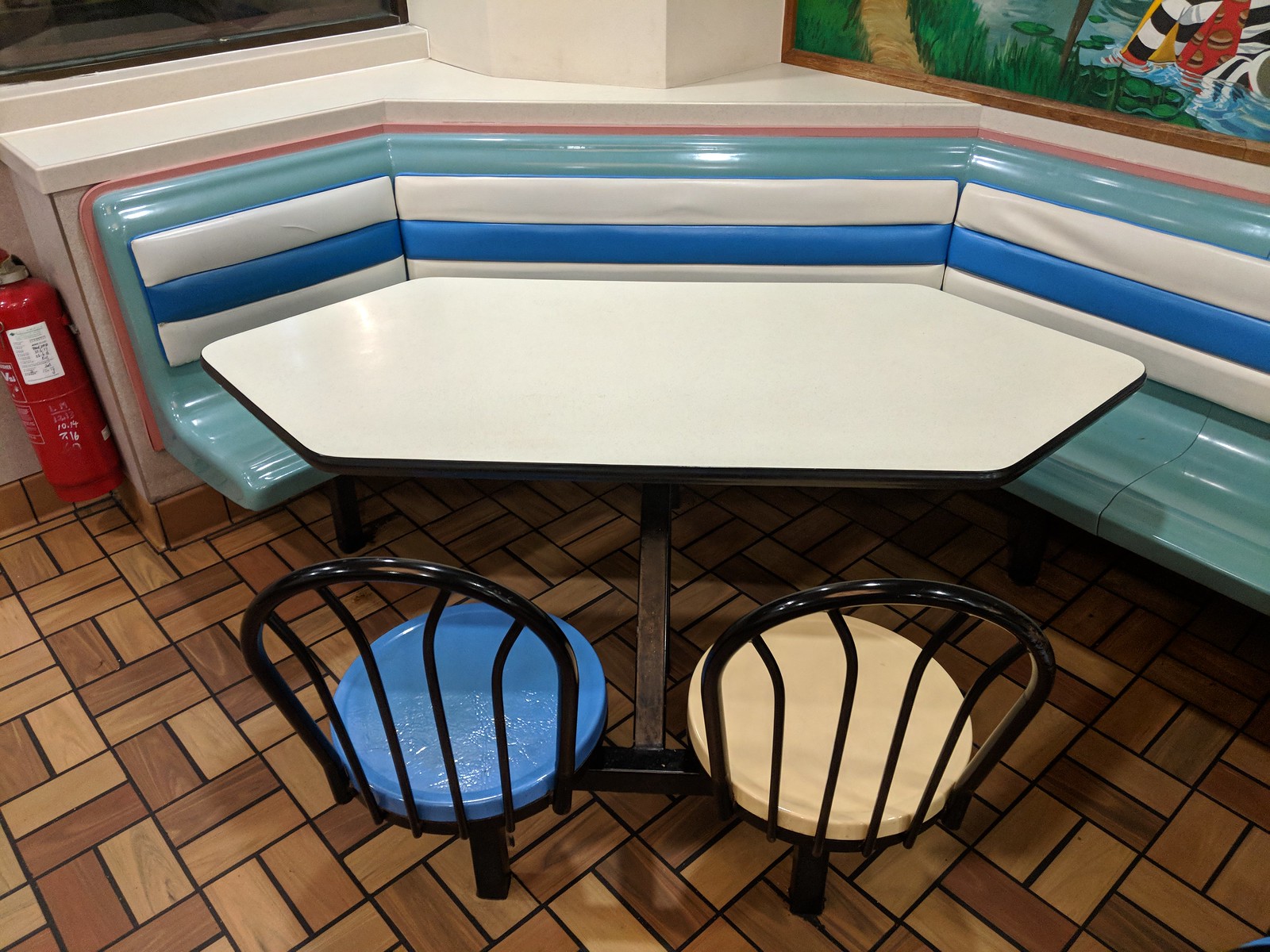The photo captures a nighttime scene inside a fast food restaurant with a clean and well-maintained dining table. The table is rectangular, oriented like a diamond, and has a distinct black trim around its white surface. Two rotating stools are attached to the table with black metal bars and are also secured to the ground for stability. One stool features a blue seat, while the other has a cream-colored seat; both have black metal backs. On the opposite side of the table, there is a bench seat with a light blue cushion. The backrest of the bench is striped, featuring a white-blue-white pattern, and has a pink salmon color outline. In the foreground and to the left, a fire extinguisher is mounted on the wall that supports the bench. The flooring is a brown rectangle pattern. Additionally, the darkened window in the top left of the frame indicates it is nighttime, and in the top right corner, a painting depicting water and a person can be seen.